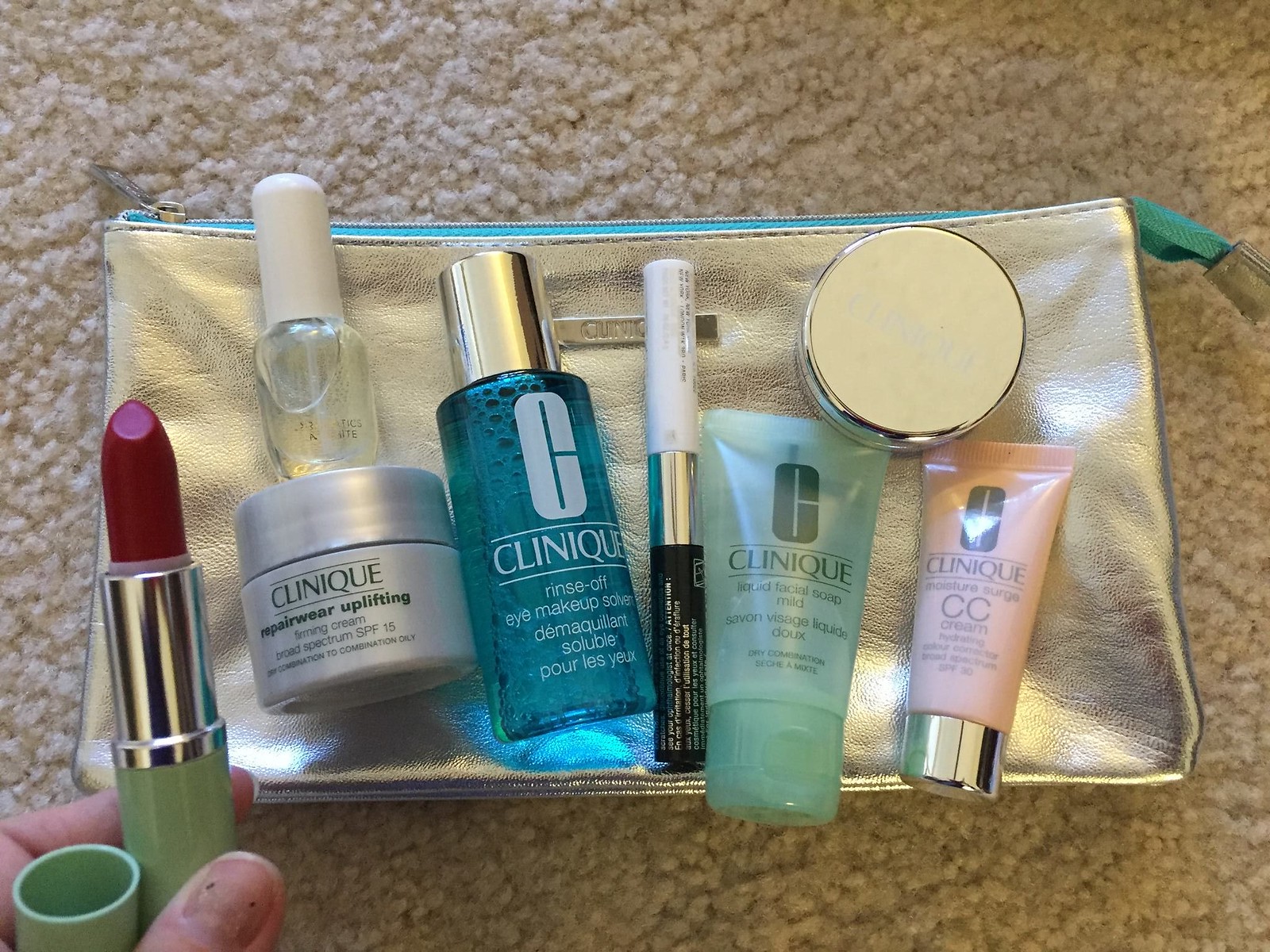The photograph features a collection of nail products and skincare items displayed on top of a compact, rectangular silver carry bag. The bag, characterized by a blue zipper, rests on a beige carpet with a normal, textured appearance, providing a neutral backdrop to highlight the items. 

In total, six products are arranged on the bag. The owner's thumb and forefinger appear at the bottom of the image, clutching a striking lipstick. This lipstick is encased in a teal tube with a chrome top, revealing a vivid red shade. 

Prominently positioned on the bag is a small tub labeled "Clinique Repairwear Uplifting Firming Cream." The text is printed in black on the silver, screw-top container. Slightly above this, a small, white-capped cylindrical tube is visible. 

Adjacent to these items is another Clinique product, a rinse packaged in a long, transparent blue plastic tube. This contains a liquid matching the tube's color and is topped with a chrome-colored cap, adding a touch of sophistication to the collection.